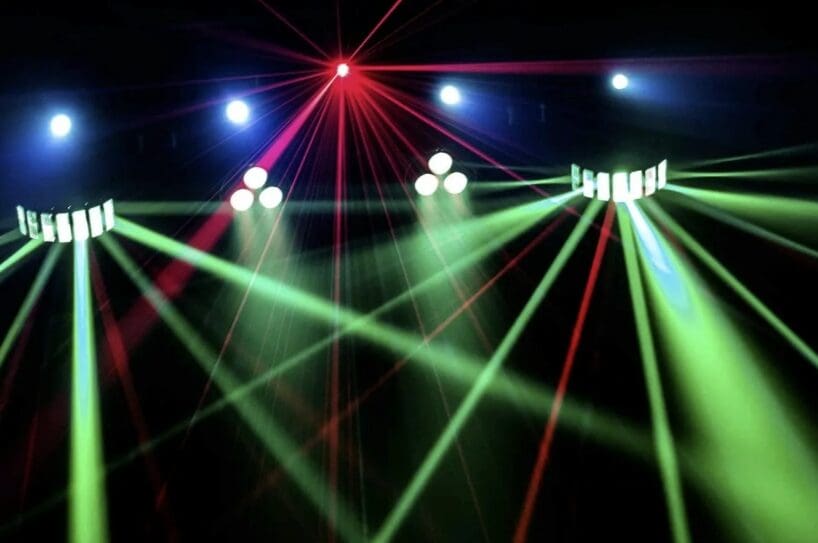The image portrays a dramatic array of concert or stage lights set against a pitch-black background. Dominating the top of the image is a row of five round, white lights spanning almost the width of the picture. Nestled among these is a striking red light, emitting vibrant red rays in all directions. Below this prominent row, there are additional lights arranged in intriguing configurations. On the left, a small row of seven vertical rectangular lights, possibly part of a circular fixture, extends just inside the left border, emitting green rays. Moving right and slightly above this, there are three distinct groups of circular lights arranged in triangular formations, each contributing their soft blue and green hues to the composition.

The green lights produce about ten concentrated beams, while the blue lights cast gentle, shadowy glows without distinct rays. The red light stands central and intense, surrounded by a halo of numerous beams. The lower top area features half-circle light formations on both sides, complementing the central row. Altogether, the image captures the vivid interplay of variously colored beams, predominantly green, red, and blue, illustrating a dynamic stage lighting setup with an emphasis on the interplay of light and shadow.